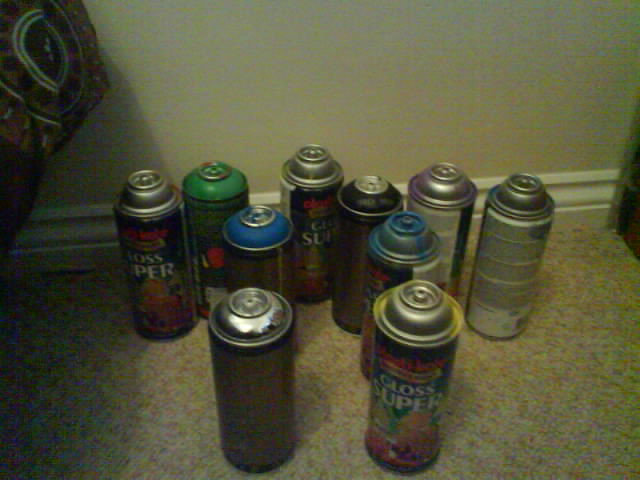In a dimly lit room with an ivory-colored wall and white baseboards, a collection of ten old spray paint cans is arranged on a multicolored carpet that resembles a Monet painting. The cans, which are various shades of blue, silver, green, black, red, and purple, are missing their spray nozzles and appear worn and rusted. Some of them are labeled "Gloss Super," although the text is difficult to read due to their age and the distant camera angle. The spray cans are positioned in a somewhat random manner: five form a loose line at the back, while four are grouped in a square shape closer to the viewer. The tops of the cans feature different colored caps, adding to the colorful yet aged appearance of the scene.